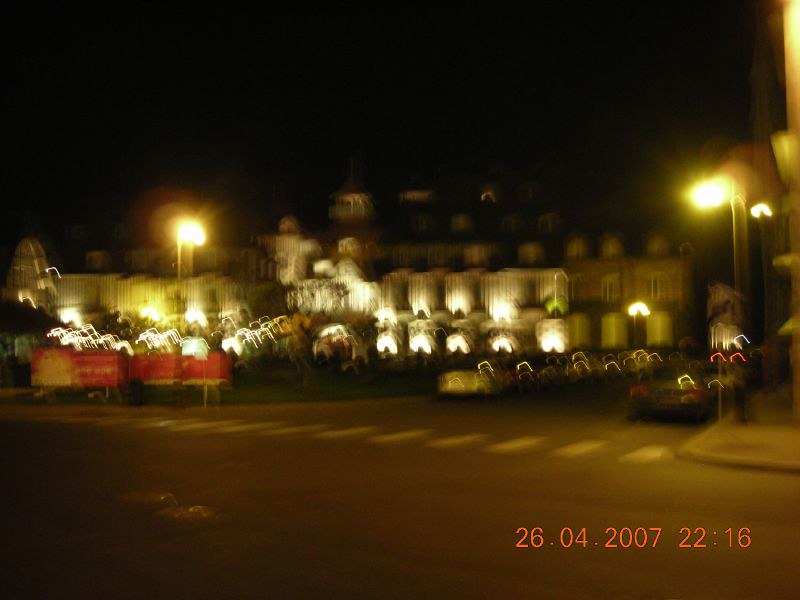This photograph, dated April 26, 2007 at 22:16, is an extremely blurry nighttime image. The main focus seems to be a large, illuminated structure that looks like a castle or perhaps a holiday display, reminiscent of Christmas decorations. The image is so out of focus that the structure's details are indiscernible, appearing as lit-up, upside-down U shapes. 

In the foreground, there is a street intersection featuring a crosswalk with the typical white rectangular markings. On either side of the intersection, there are cars parked, possibly a black car and a gray car, although the blur makes it hard to confirm. The street is illuminated by bright, yellowish-orange lights, with one streetlight on the left and another on the right. There is also a red sign at the bottom left of the image, but its text is unreadable due to the blurriness. Overall, the photograph's extreme blur makes it difficult to discern precise details of the scene.